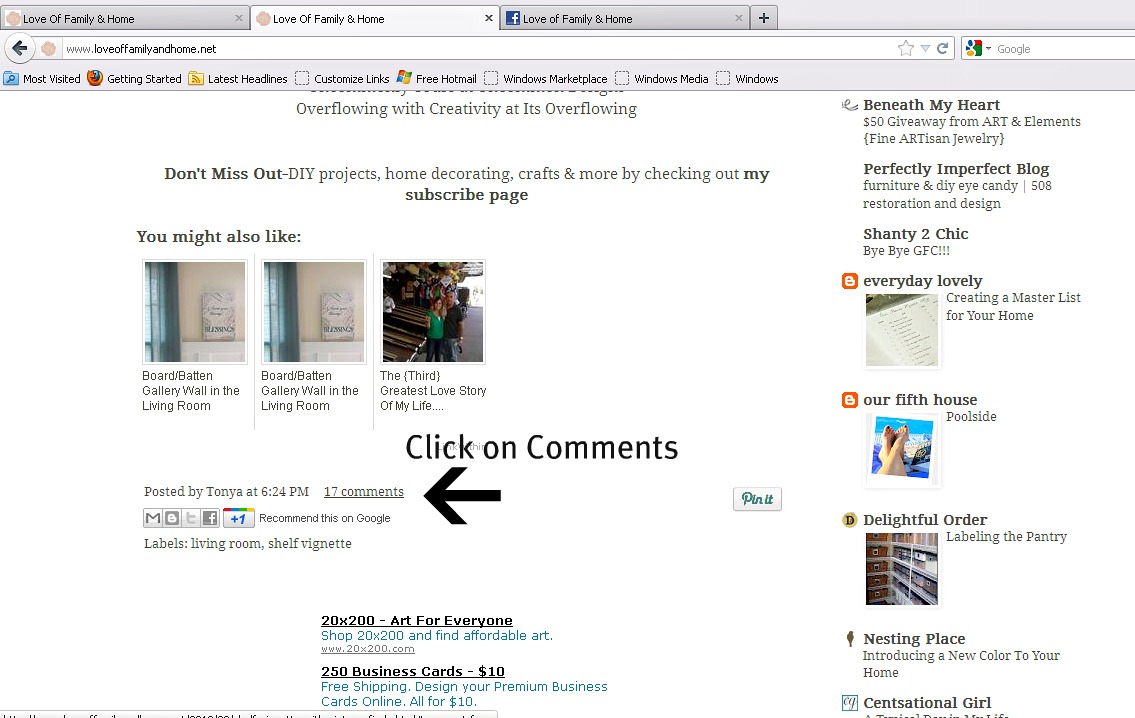The image is a detailed screenshot of a family-themed blog website viewed on a computer screen. At the top of the browser window, three tabs are open, all featuring 'Love of Family and Home' – two from the same site and one from its Facebook page. The URL displayed is www.loveoffamilyandhome.net.

The webpage's navigation bar includes options like Menu, Most Visited, Getting Started, Latest Headlines, Customized Link, Free Hotmail, Windows Marketplace, Windows Media, and Windows. The site exudes a creative vibe, inviting visitors not to miss out on DIY projects, home decorating ideas, crafts, and more by checking out the subscription page.

Below the header, a section titled 'You might also like' showcases small icons with accompanying texts, such as 'Board & Batten Gallery Wall in the Living Room' and 'The Third Greatest Love Story of My Life.' There's a prominent arrow directing users to click on 'Comments.' A post by Tanya is shown, timestamped at 6:24 PM with 17 comments underneath. 

The right-hand sidebar features various blog names and offerings like 'Beneath My Heart,' a '$50 giveaway,' 'Perfectly Imperfect Blog,' 'Furniture and DIY Eye Candy,' 'Shanty 2 Chic,' 'Bye Bye GFC,' 'Everyday Lovely,' 'Our 5th House,' 'Delightful Order,' and 'Nesting Place.'